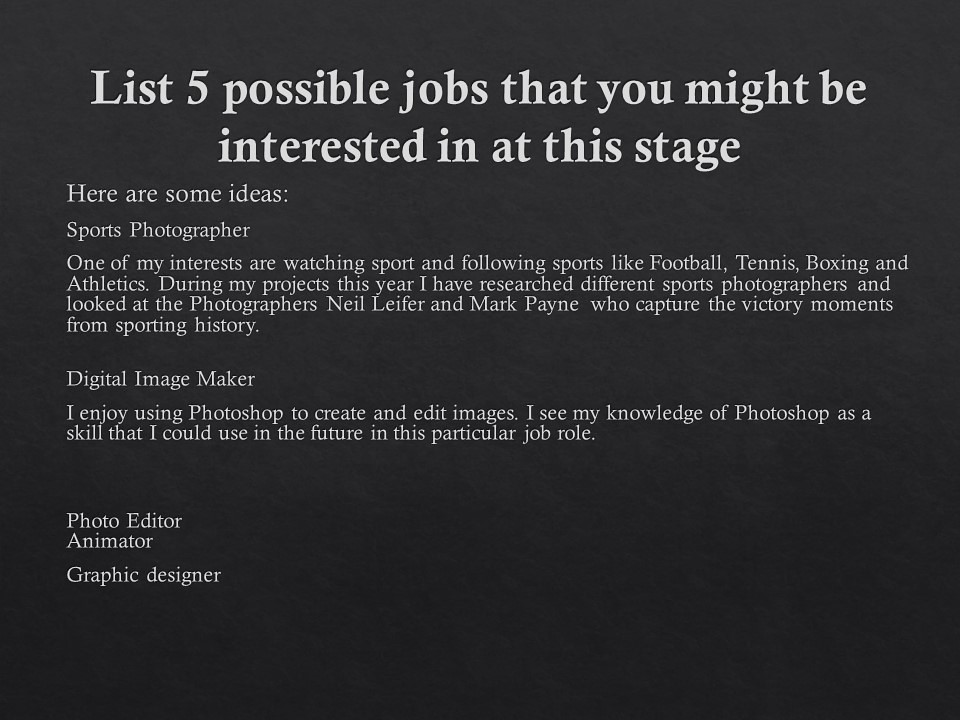The image is a predominantly black presentation slide, subtly transitioning from dark gray at the top to black at the bottom, possibly featuring a very fine texture. It contains large white text at the top, which serves as the heading and reads, "List five possible jobs that you might be interested in at this stage." Below this, smaller white text introduces possible job ideas. The first suggestion is "Sports Photographer," with a brief explanation stating: "One of my interests is watching and following sports like football, tennis, boxing, and athletics. During my projects this year, I have researched different sports photographers and looked at the works of Neil Leifer and Mark Payne, known for capturing iconic victory moments in sporting history." The next job suggestion listed is "Digital Image Maker," followed by an explanation: "I enjoy using Photoshop to create and edit images. My knowledge of Photoshop is a skill that I could leverage in this job role." Additional job roles mentioned are "Photo Editor," "Animator," and "Graphic Designer."